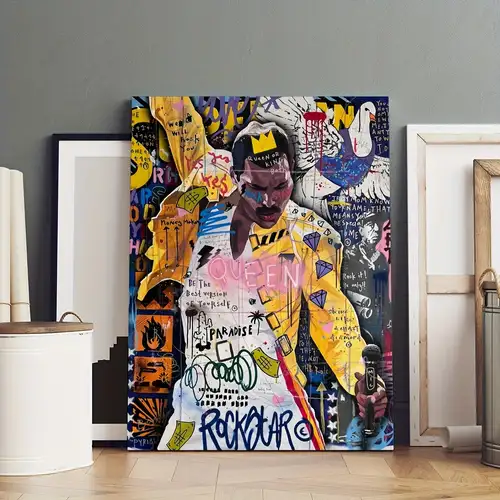This photograph captures a large, vibrant piece of modern art, roughly 10 feet tall, leaning against a light gray wall. The centerpiece of the artwork is a collage featuring the iconic singer Freddie Mercury, depicted facing forward and looking down. He is dressed in a white outfit highlighted by a bright yellow jacket, and holds a microphone in his left hand. His right arm is outstretched upwards. Atop his head rests a yellow crown, and the word "Queen" is prominently displayed in pink text across his torso. The painting's background is dense with various graffiti-like elements, small drawings, and random letters, giving it a layered, textured feel. A white dove adorned with a blue vest is positioned in the upper right corner of the artwork. The word "Rockstar" is inscribed in blue graffiti at the bottom of the piece. Surrounding this central art piece, the setting reveals a brown-tiled floor and several other framed artwork pieces, some turned towards the main painting and others away, implying a storage or preparation area possibly for hanging these artworks. Additionally, rustic farmhouse-style baskets and scrolls tied with rubber bands are visible, enhancing the eclectic atmosphere. A small, white container with a brown lid tied with a rope sits nearby, adding to the detailed setting of the scene.